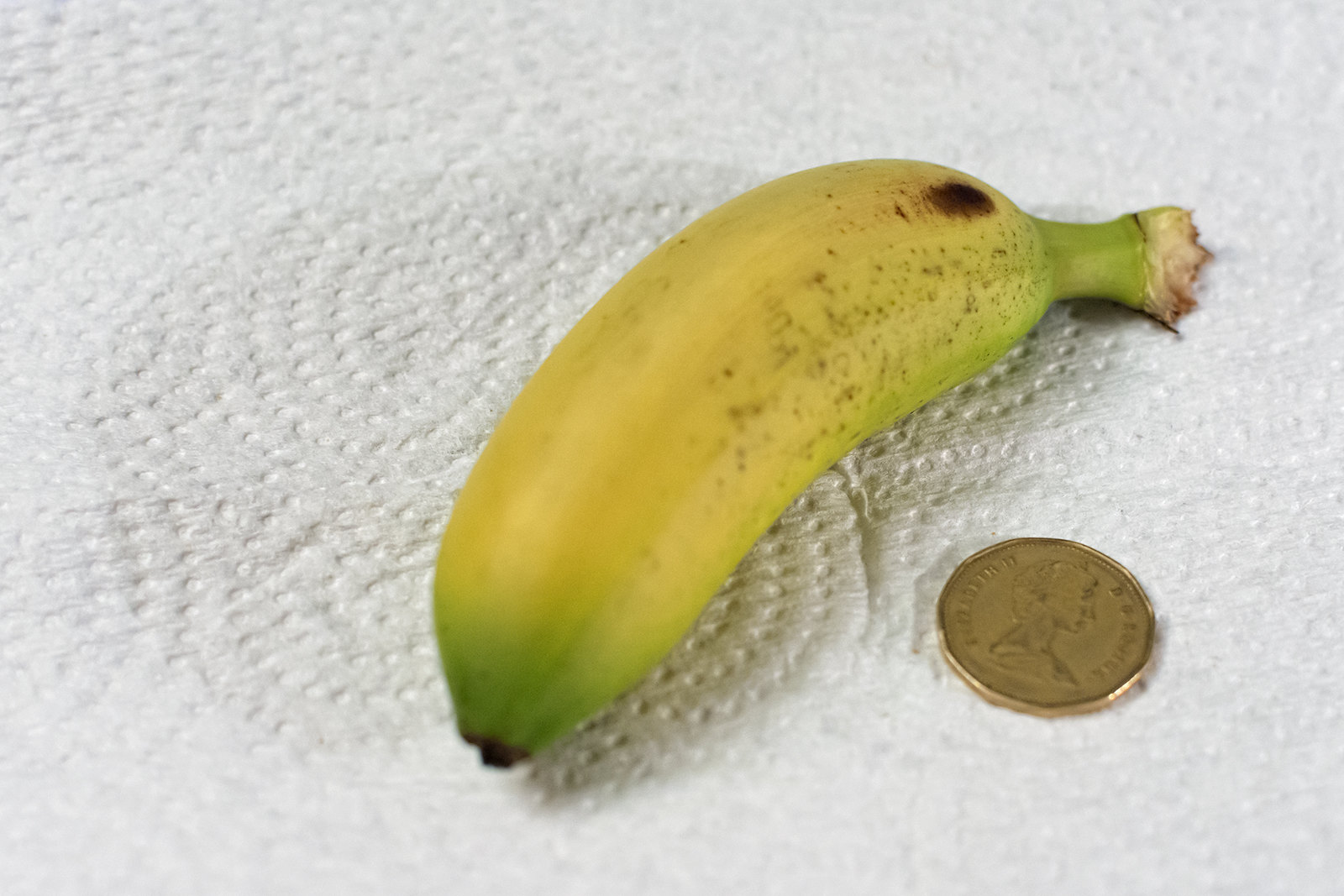Resting on what seems to be a paper towel, another sheet of paper towel can be seen underneath, marked with numerous dots and indents. On the middle right of the image, there is a notably plump banana. Its stem is green, indicating where it was once connected to a bunch. The banana itself displays a gradient of colors: the tip on the left is dark green, transitioning to mostly yellow with some brown speckles in the middle, and culminating in a large brown spot on the right side. 

Positioned beneath the banana, there is a coin, presumably made of brown copper. The coin features text along its circumference, though the exact wording is difficult to discern. At the center of the coin, there is a carving of a person’s side profile, showcasing distinct curls at the top of the head which are highlighted by light around the edges. The profile shows shadowing in the middle, suggesting the illumination is primarily from the right side. The coin, circular by nature, is designed with multiple sides creating a faceted look with edges that appear worn, indicative of weathering.